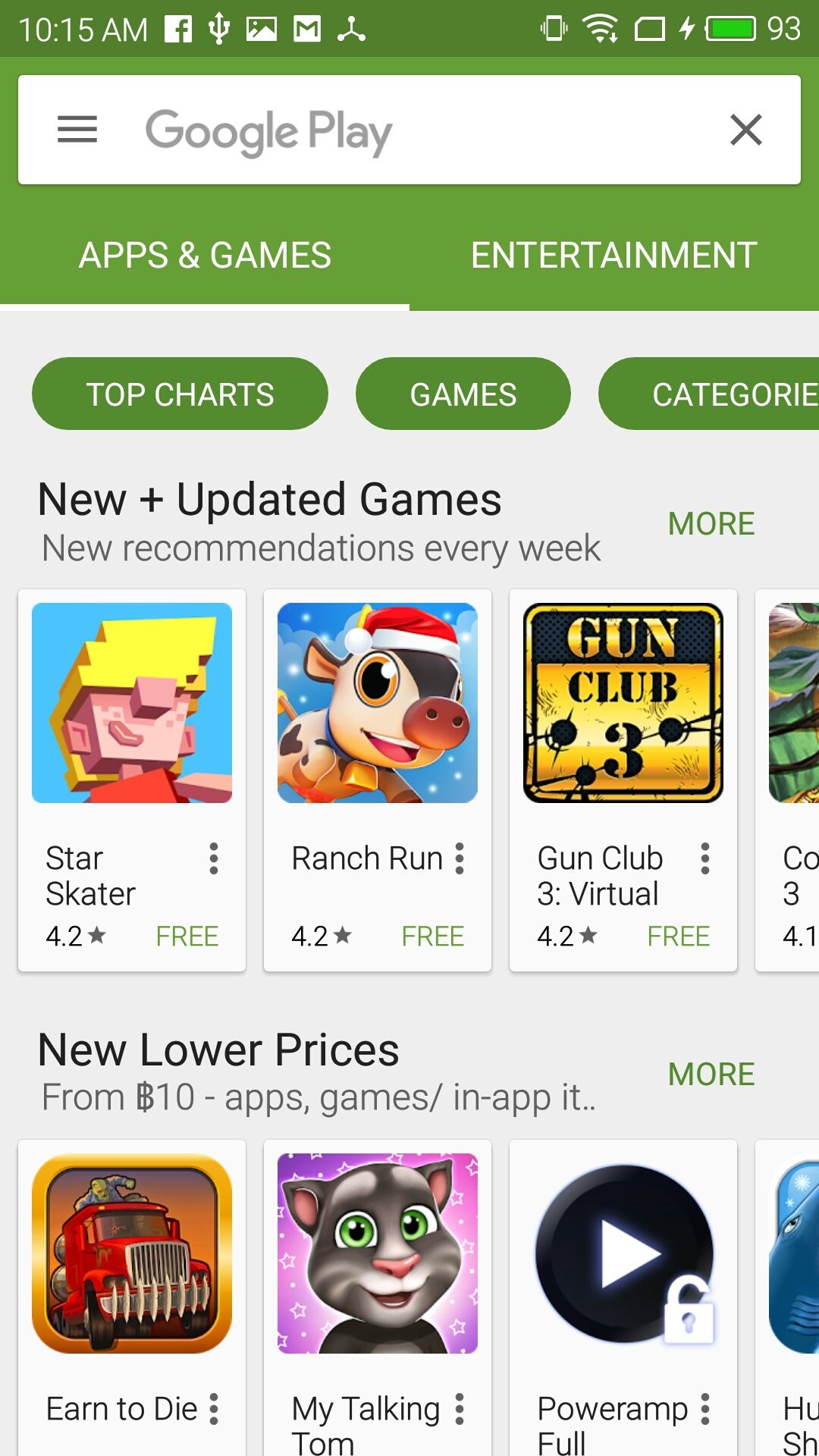The image is a portrait-oriented screenshot from a phone displaying the Google Play Store interface. The top section of the image features a dark green border containing various white icons. From left to right, these icons include: the time "10:15 AM," a white box with a green "F" representing Facebook, a Trident-like icon for sharing, an image icon, a Google Mail icon, an unidentified icon with three points (two at the bottom and one at the top in the middle), a vibrate phone icon, a fully-filled Wi-Fi connection meter, a fast charging icon indicated by a lightning bolt, and a battery icon showing a 93% charge.

Below the dark green border is a white Google Play search box. Beneath the search box are two options in a light green background with white text: "Apps & Games" and "Entertainment." Further down, there are three light green bubbles with white text labeled "Top Charts," "Games," and "Categories."

The midsection of the screenshot displays a section titled "New and Updated Games," with a subheader stating "New Recommendations Every Week." This section showcases games such as "Star Skater," "Ranch Run," "Gun Club 3," and "Virtual." Another section is highlighted underneath with a header that says "New or Lower Prices from 10 Bitcoin," featuring titles like "Earn to Die 2" by Talking Tom and "Power Ample."

The image overall shows search results and suggested applications from the Google Play Store.